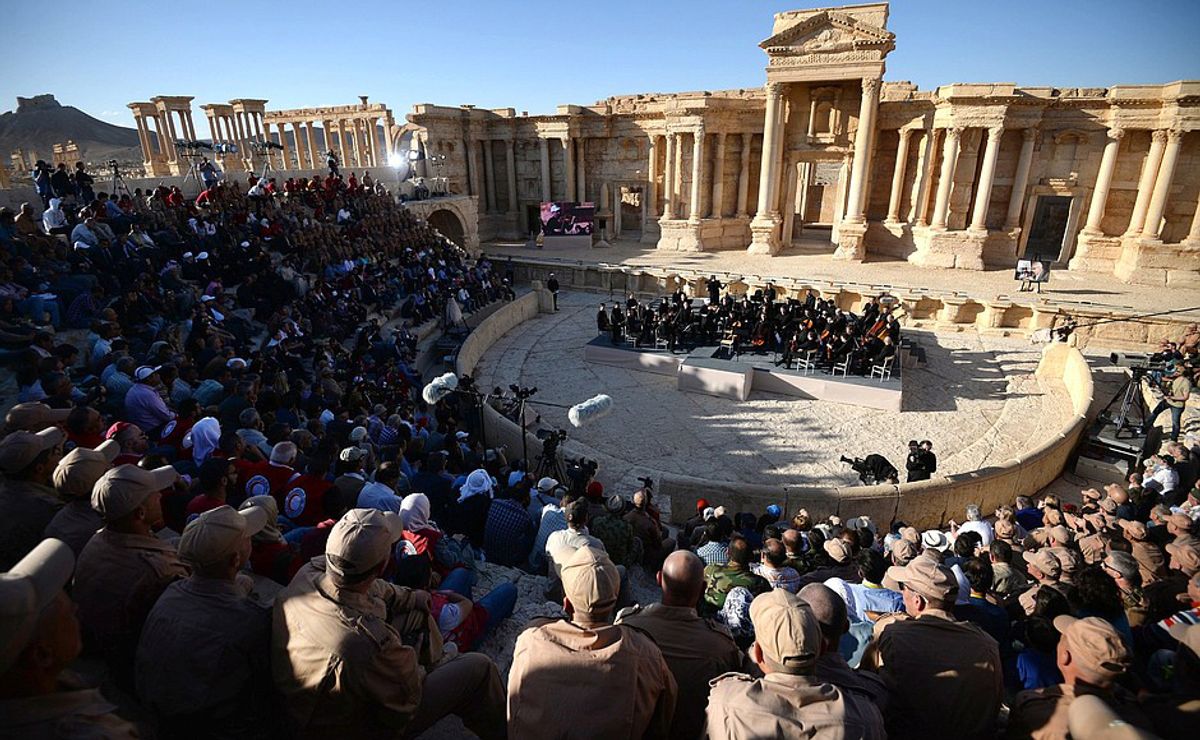In the image, a large crowd of over a hundred people is seated in an ancient Colosseum, possibly from Ancient Rome or Greece. The amphitheater's ruins, complete with grand columns and intricate architectural details, form a dramatic backdrop to the scene. The spectators, many of whom wear brown shirts and matching ball caps, possibly indicating a group or military presence, are all intently focused on a performance taking place below. On the stage at the center of the arena, musicians dressed in black play their instruments, which could be violins or similar. Cameras and microphones are visible among the crowd, capturing the event. Behind the amphitheater, a tall mountain rises majestically, and the clear, sunny sky adds to the atmosphere of a significant and well-attended event in this historic location.